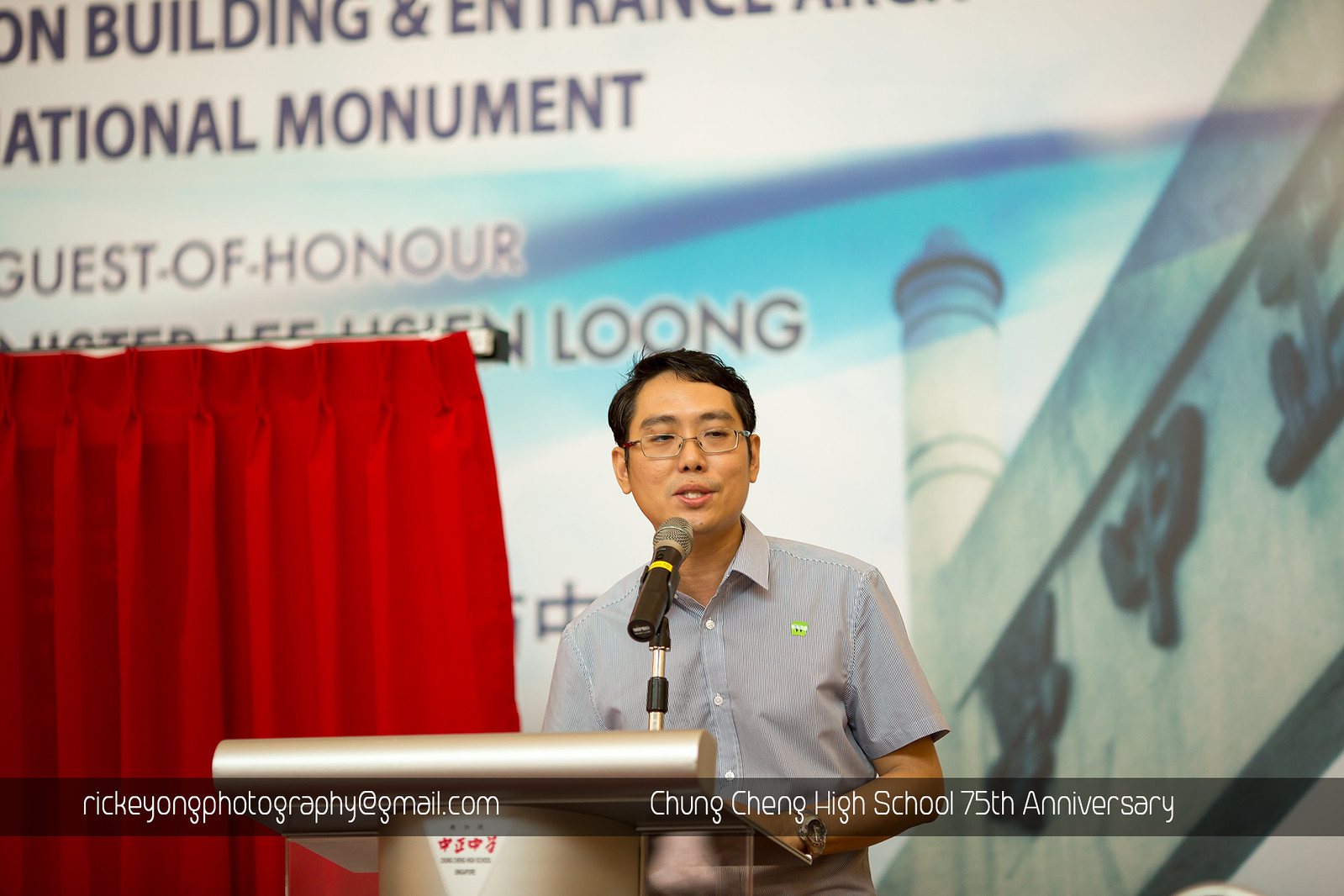In this image, a man with short black hair and glasses is standing behind a metallic podium, located centrally at the bottom of the frame, where he appears to be delivering a speech. He is dressed in a light-colored button-down shirt adorned with a symbol on the left chest area. Positioned directly in front of him, a microphone is raised to his face. A red curtain, hanging on a white horizontal rod, is visible to his left, extending from the middle to the bottom of the image. 

The backdrop features a large screen displaying an image of a building and partially obscured text. The decipherable text at the top reads "National Monument" and further down "Guest of Honor," although some portions are cut off. Surrounding the screen is a blend of colors, including white, black, dark blue, light blue, red, gray, silver, yellow, neon, and green. The lower portion of the image also includes a border with white lettering. On the left, it reads "rickeyongphotography@gmail.com," while on the right it announces "Chong Cheng High School 75th Anniversary." The setting appears to be indoors during a school anniversary celebration.